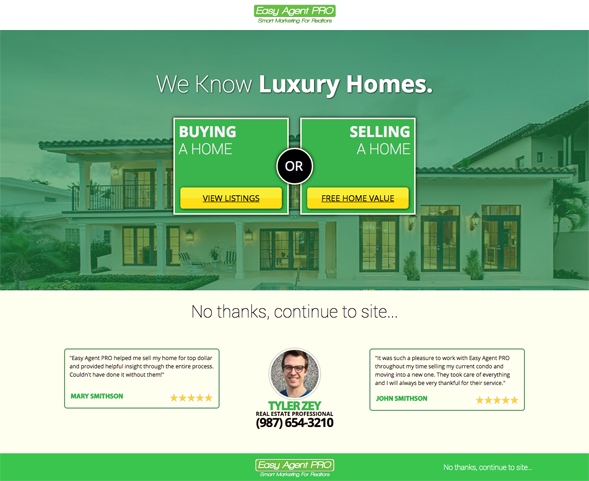The image showcases the homepage of a website called Easy Agent Pro. At the top center of the page, the website's title is prominently displayed in white lettering against a green banner. Below the banner, there's a large, green-tinted image of a property, emphasizing the website's green theme. Overlaid on this image is the text "We know luxury homes," with "Luxury homes" in bold white letters and "We know" in finer white letters.

Beneath the featured image, there are two green boxes with fine white borders. The first box, labeled "Buying a home," features "Buying" in bold white lettering. Below this text is a yellow button with black text that reads "View listings." The second box, to the right, is similarly styled but is labeled "Selling a home," with "Selling" in bold white letters. Underneath this text is a yellow button that reads "Free home value" in black and is underlined. 

Between these two boxes is a prominent black dot with a white outline and the word "OR" written in white at the center. Below this section, there is an option to "No thanks, continue to site" displayed against a white background. The lower part of the page features several testimonials on both the left and right sides, showcasing client experiences and feedback.